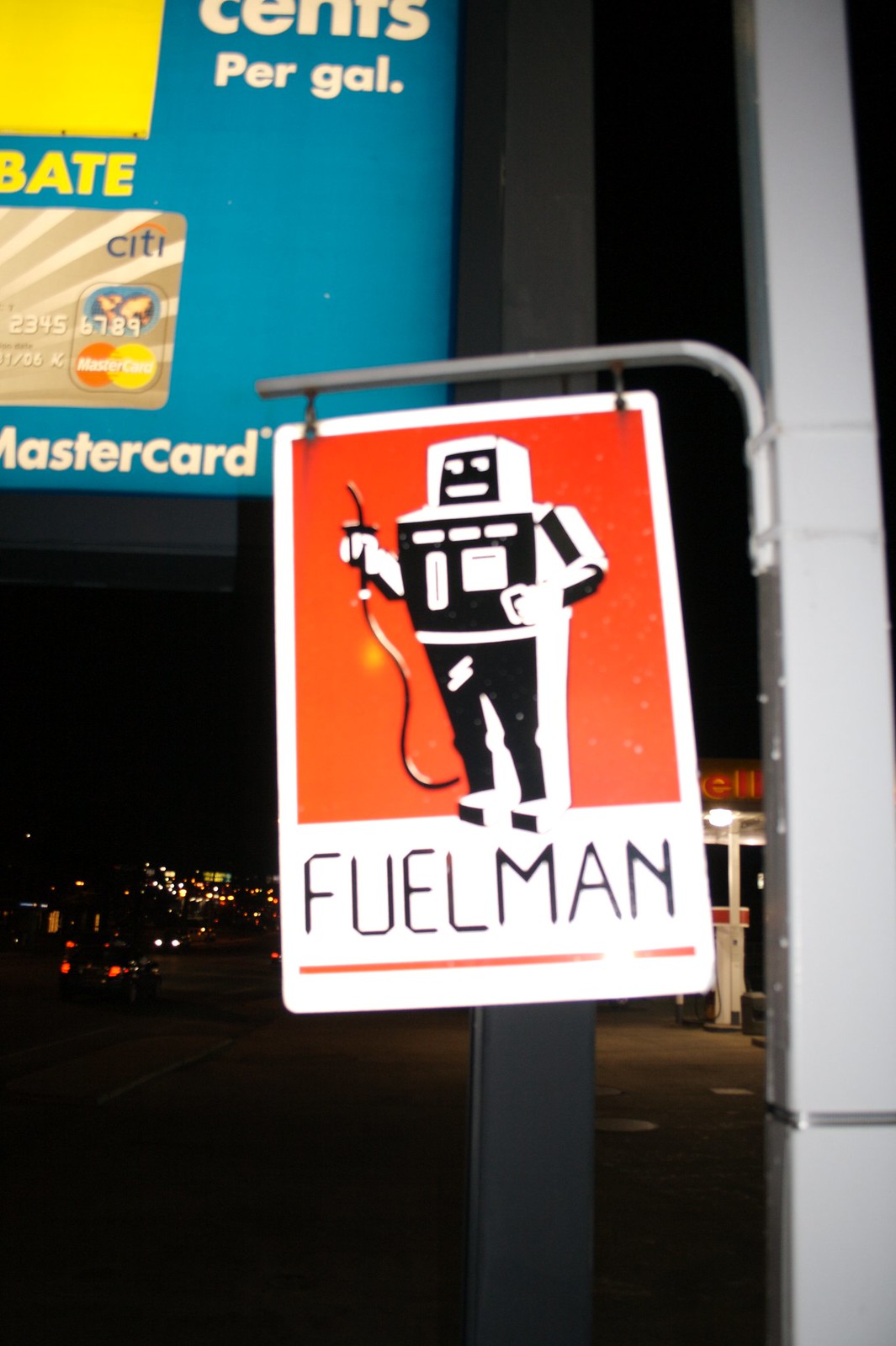This photograph features a street sign prominently displayed on a tall metal pole. The main sign is a white rectangle with an orange square in the center, featuring a black and white robot holding a fuel nozzle, visually representing a gas pump. Below the robot, the text reads "Fuelman," identifying the robot as the gas station's mascot. Above this main sign, there's another blue sign, partially visible, indicating fuel prices with the mention of "cents per gallon," and it includes an image of a credit card, suggesting that MasterCard payments are accepted. The photo is taken at night, with city lights visible in the distance, hinting at an urban setting.